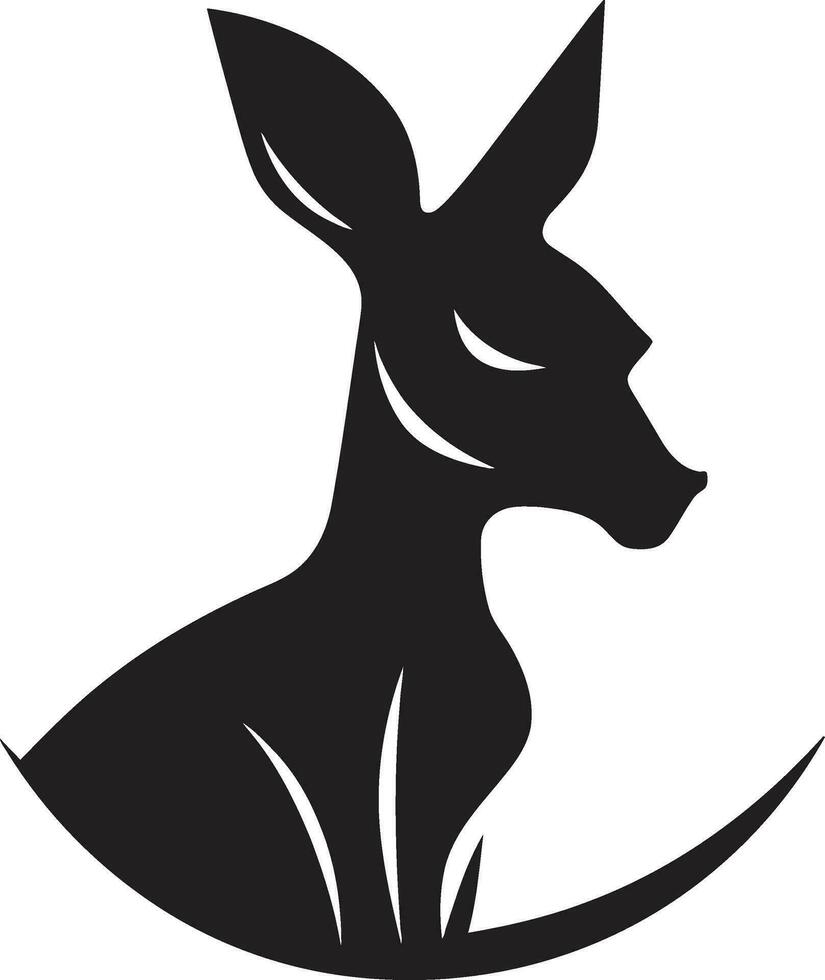The image is a professional, high-resolution digital logo featuring a minimalistic black silhouette of a deer against a white background, possibly designed for an organization or company. The deer, which appears to be female due to the absence of antlers, is depicted in a right-facing profile view. The intricate use of white space highlights details such as the eye slit, parts of the ear, and areas around the neck and chest. The design showcases only the deer's head and upper torso, ending in a rounded arc at the bottom, reminiscent of a crescent moon or a rocking chair curve. The image lacks any contextual elements, enhancing its stark, simplistic aesthetic.